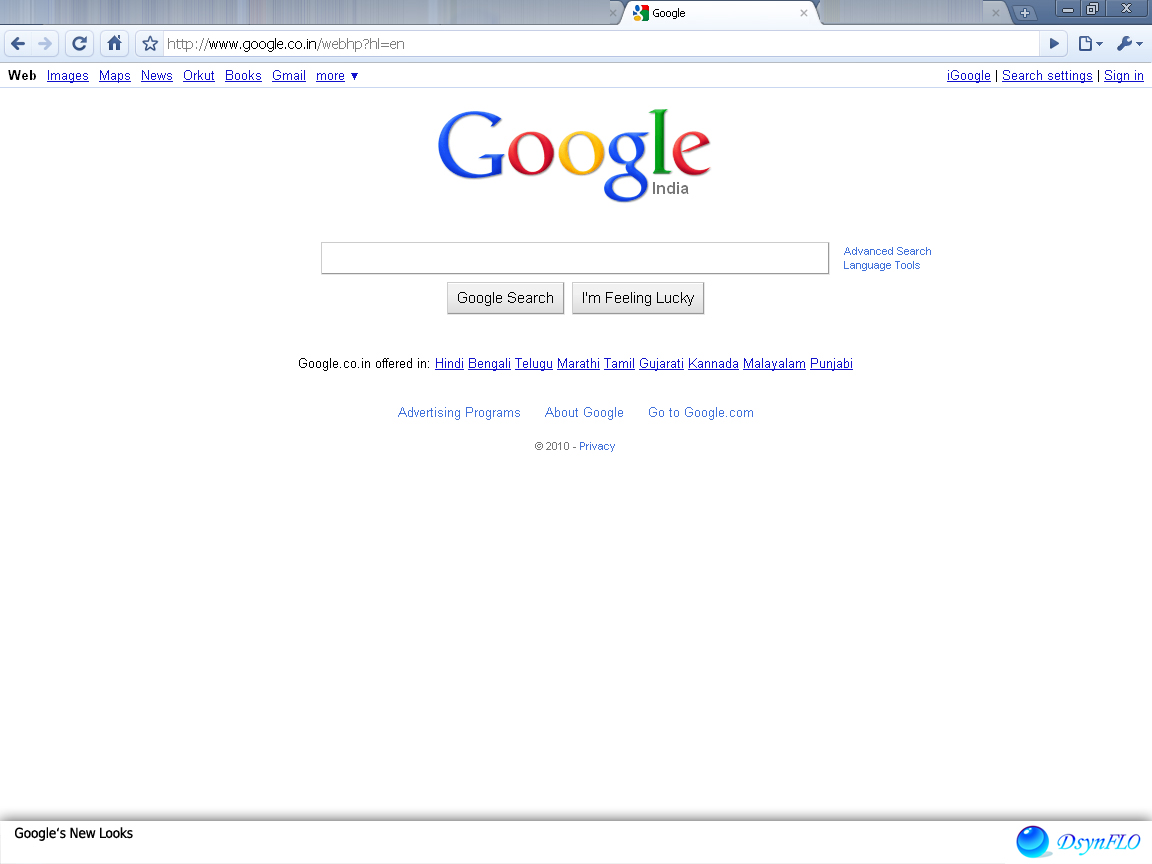The image showcases a computer monitor displaying the Google homepage. Specific details include:

- The Google tab is open, with the URL "www.google.co.in" visible in the address bar.
- Navigation elements highlighted include a left-facing arrow, a right-facing arrow, a refresh button, a home button, and a star icon.
- Adjacent to the address bar are two icons with drop-down arrows: a document icon and a wrench icon.
- Directly below the address bar, several tabs are visible: "Web" (the current tab), "Images," "Maps," "News," "Orkut," "Books," "Gmail," "More" (with a drop-down arrow), "iGoogle," "Search settings," and "Sign in."
- The central part of the page features the iconic Google logo with "India" written beneath it, followed by a prominent search bar, options for "Advanced search" and "Language tools."
- Below the search bar, there are two grey buttons: "Google Search" and "I'm Feeling Lucky."
- Further down, "www.google.co.in" is shown, with the site offered in various Indian languages: Hindi, Bengali, Telugu, Marathi, Tamil, Gujarati, Kannada, Malayalam, and Punjabi.
- The footer of the page includes links to "Advertising programs," "About Google," and an option to "Go to www.google.com." It also shows "Copyright 2010" and "Privacy."
- On the left side of the footer, a note states "Google's new look."
- On the right side of the footer, there appears to be an icon resembling a marble, followed by the text "D-S-Y-N-F-L-O," with "F-L-O" capitalized.